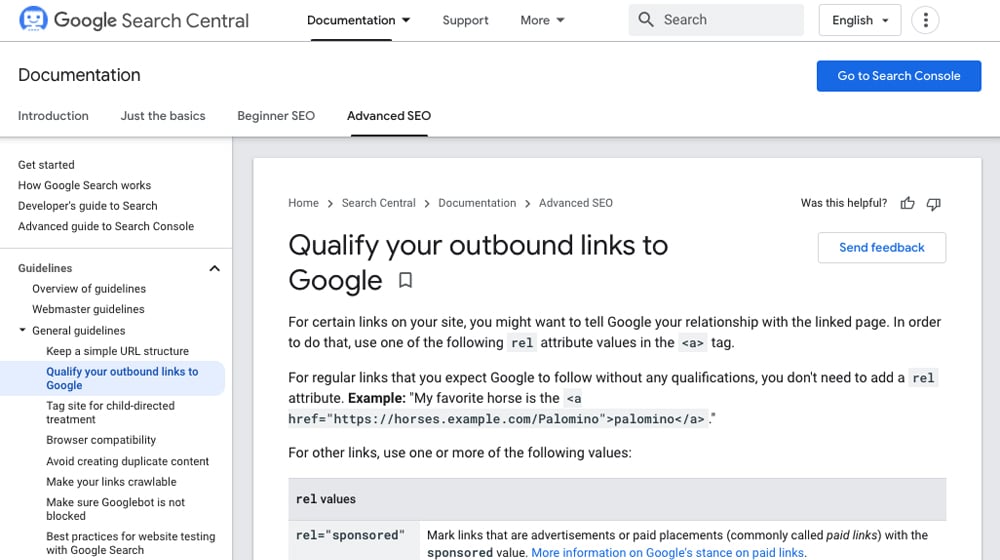Screenshot of the Google Search Central Website

This detailed screenshot of the Google Search Central website is taken from a monitor and showcases the back end interface designed for webmasters to fine-tune their search settings.

**Header Section:**
- **Top Left Corner:** A blue circle featuring a small white robot icon is displayed, followed by “Google Search Central” in black text.
- **Top Center:** The navigation menu includes “Documentation” (selected and underlined by a black bar), “Support,” and “More” (both accompanied by down arrows for dropdown options).
- **Top Right Corner:** Features a search bar with a gray magnifying glass icon and a drop-down menu for language selection, currently set to English. To the right is a circle with three vertical black dots.

**Main Content Area:**
- **Left Column:** Labeled “Documentation” with three primary menu labels:
  - **“Introduction”**
  - **“Just the Basics”**
  - **“Beginners SEO”**
  - **“Advanced SEO”** (all in bold black text with a black line underneath them)
- **Far Right Column:** Contains a blue rectangular button with white text that says "Go to Search Console."

**Primary Section Heading:**
- Outlined by a heavy gray border, the center area is white with labels:
  - **Upper Left Corner:** "Home," "Search Central," "Documentation," "Advanced SEO," and "Qualify Your Outbound Links to Google" (in bold black text).

**Interactive Elements:**
- **Upper Right Area:** A prompt "Was this helpful?" accompanied by thumbs up and thumbs down icons for feedback.
- **Below:** A white rectangular button labeled "Feedback" in blue text.

**Additional Information Column (Left Side):**
- Subheadings and navigation options include:
  - **“Get Started”**
  - **“How Google Search Works”**
  - **“Developer's Guide to Search”**
  - **“Advanced Guide to Search Console”**
  - **“Guidelines” and “General Guidelines”** (listed in black text).

This comprehensive screenshot demonstrates the layout and features of Google Search Central's webmaster interface, helpful for those looking to improve and manage their search engine strategies.